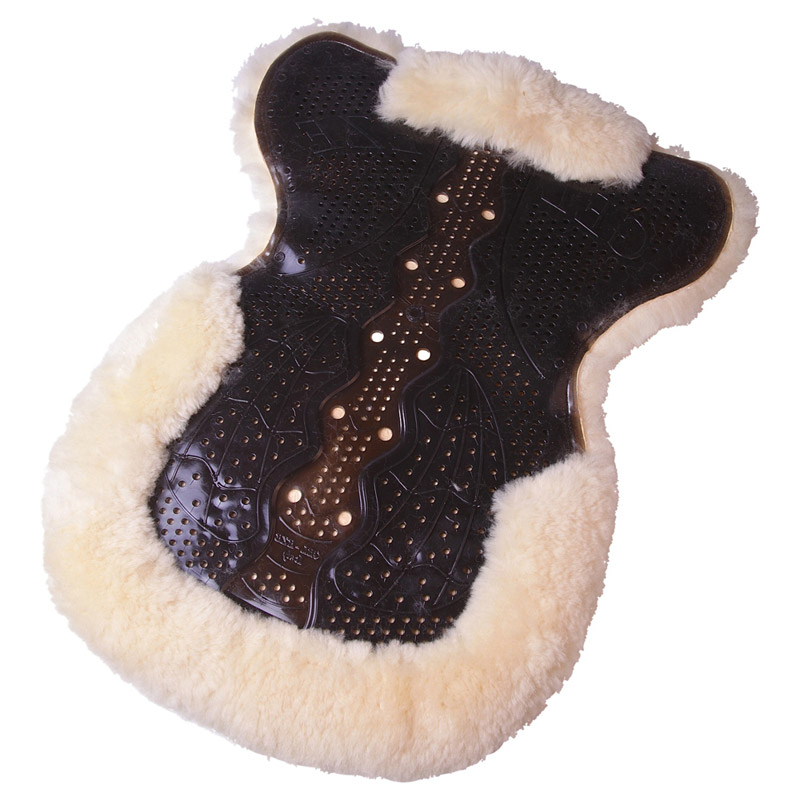This photograph features an intricately designed dark brown leather item that resembles a saddle or possibly a guitar head. The central structure of the piece has ridges creating different shaped sections, each adorned with numerous small holes. The leather is framed by a prominent border of off-white fur, which appears softer and thicker around the top and bottom, and thinner along the sides. Adding to the uniqueness, the middle section of the item includes a medium wood piece, reminiscent of a guitar fretboard, with five light-colored circles on the side and smaller circles aligned in the center. The combination of materials and patterns gives the object a highly detailed and textured appearance, blurring the lines between functional design and artistic craftsmanship.